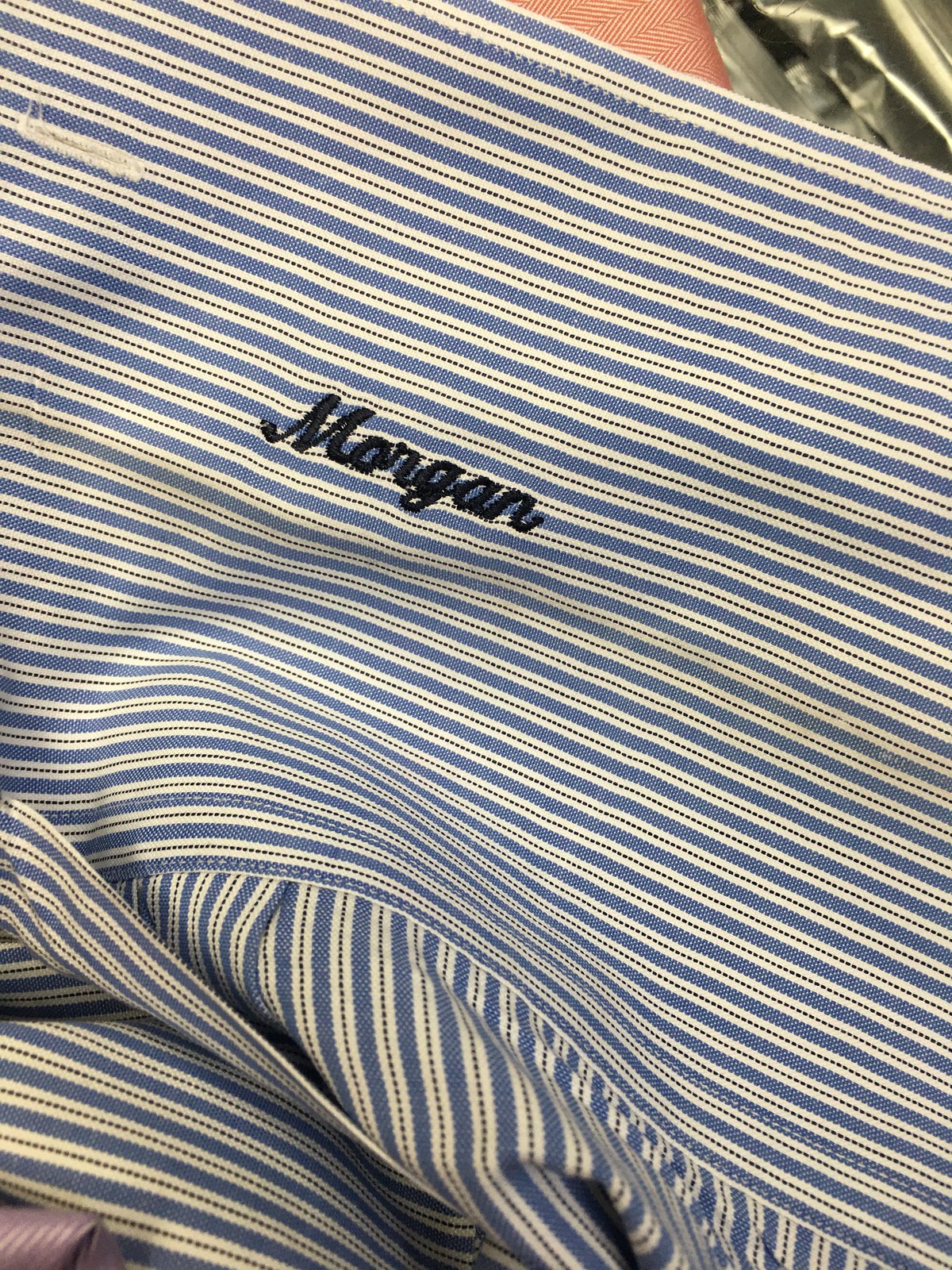The image depicts a meticulously crafted piece of textile, possibly a shirt or a bag, adorned with a personalized stitched name. The fabric features a repeating sequence of horizontal stripes in blue, white, dotted black, white, and blue, creating a visually appealing layered pattern. Positioned prominently in the center is the name "Morgan," elegantly embroidered in black cursive thread. The careful stitching and detailed pattern suggest a high level of craftsmanship. The textile item is neatly laid out on a flat surface, enhancing the clarity and visibility of the intricate details and personalized elements.